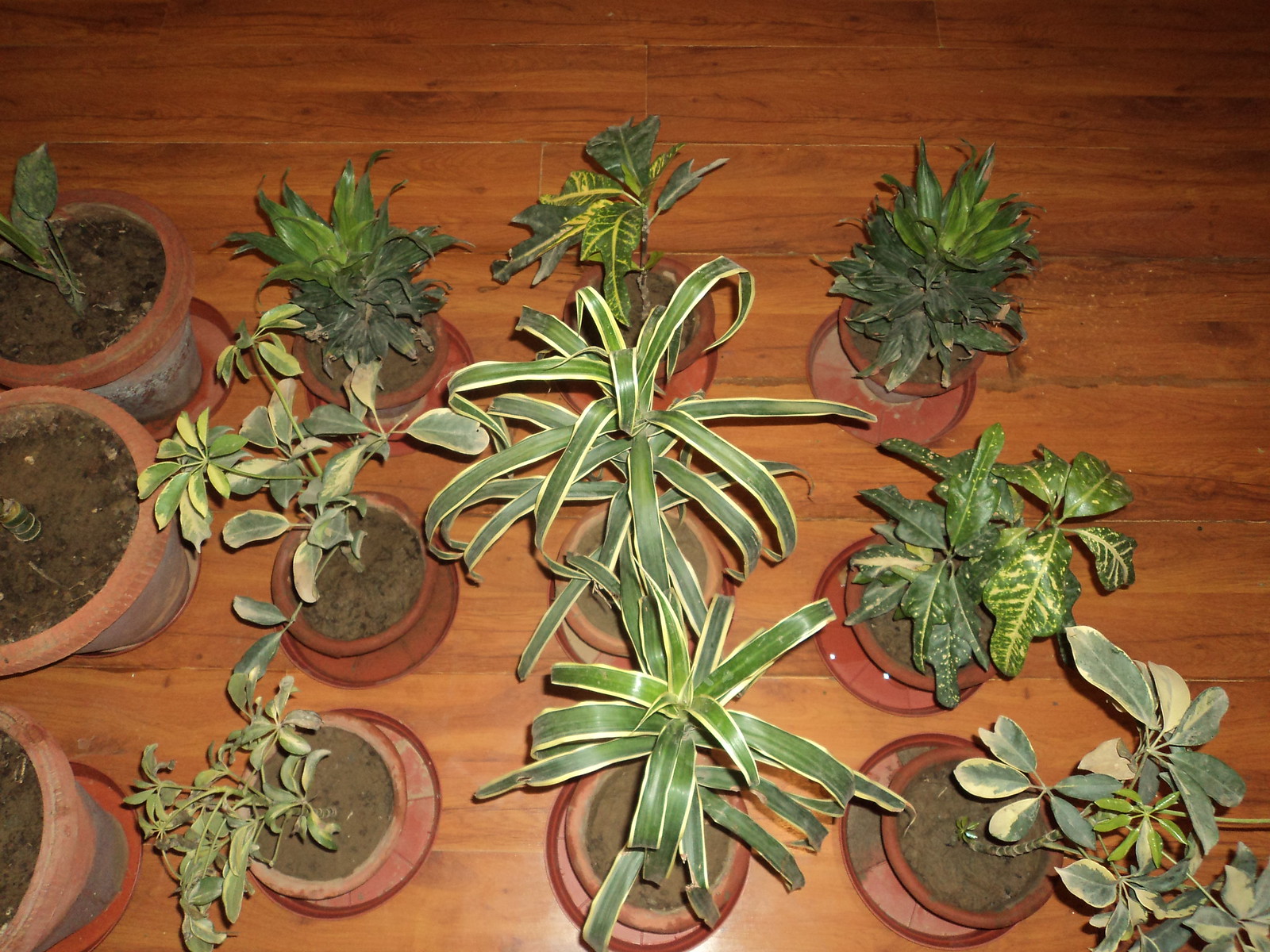This vibrant, color photograph presents a top-view angle of sixteen houseplants arranged in a 4x4 matrix on an orangey-brown wooden surface. Each plant is housed in a terracotta pot of varying sizes. The leftmost column displays minimal foliage, while the second column from the left shows plants with slightly more leaves. The central columns prominently feature two large spider plants towards the middle and bottom, accompanied by a smaller plant with wider leaves at the top. The rightmost column contains stockier, smaller plants, with the bottommost one flaunting greyish leaves that seem to face the bottom corner of the picture. Although most plants appear healthy and lush, a few show signs of dryness. The scene is illuminated with artificial lighting, indicating indoor placement, though it's ambiguous whether these plants are exclusively indoor or temporarily indoors. The warm, reflective surface beneath the pots, possibly hardwood flooring, enhances the earthy charm of this meticulously arranged botanical display.